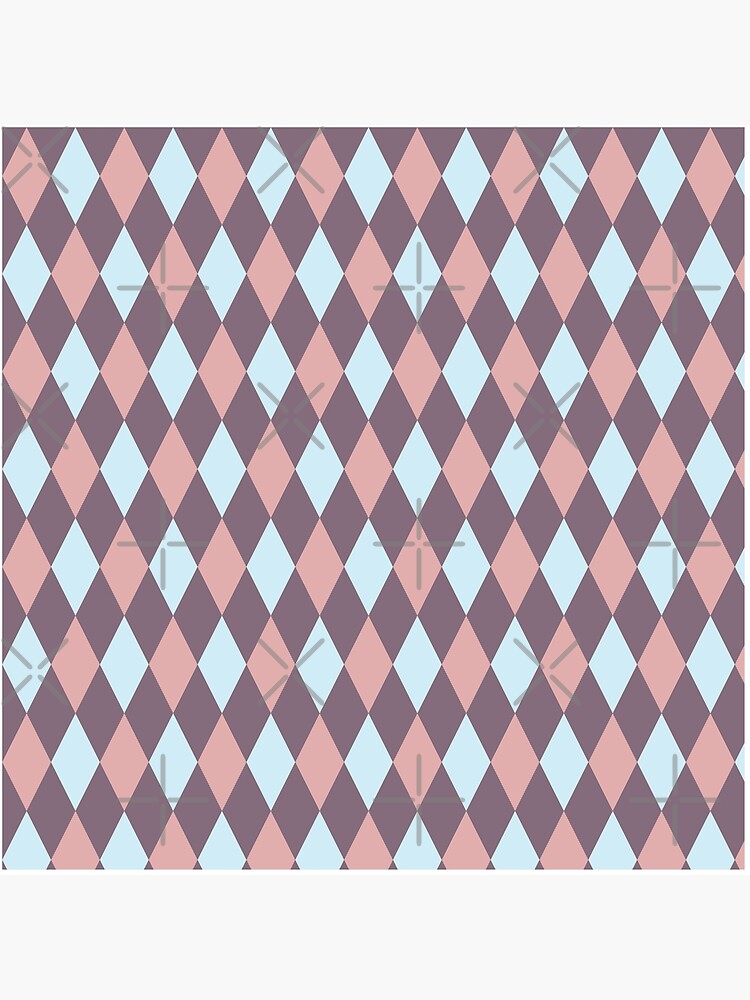This image depicts a digital stock pattern characterized by a series of diamond shapes that run diagonally in both directions, creating an overlapping X formation. The primary colors in the pattern include light salmon pink, baby blue, and a dark gray with subtle red undertones. These diamond shapes are arranged against a light blue background and separated by thin gray intersecting lines, giving a textile-like appearance that could be seen on wallpaper or fabric, such as a sweater or sock. The design, which includes alternating shades of pink and blue with intermittent white spaces, evokes a traditional or preppy style and is set within a square format that could aesthetically cover a wall, making it suitable for spaces like a bedroom or living room. The pattern is visually reminiscent of something one might encounter in a vintage diner or similar retro setting.